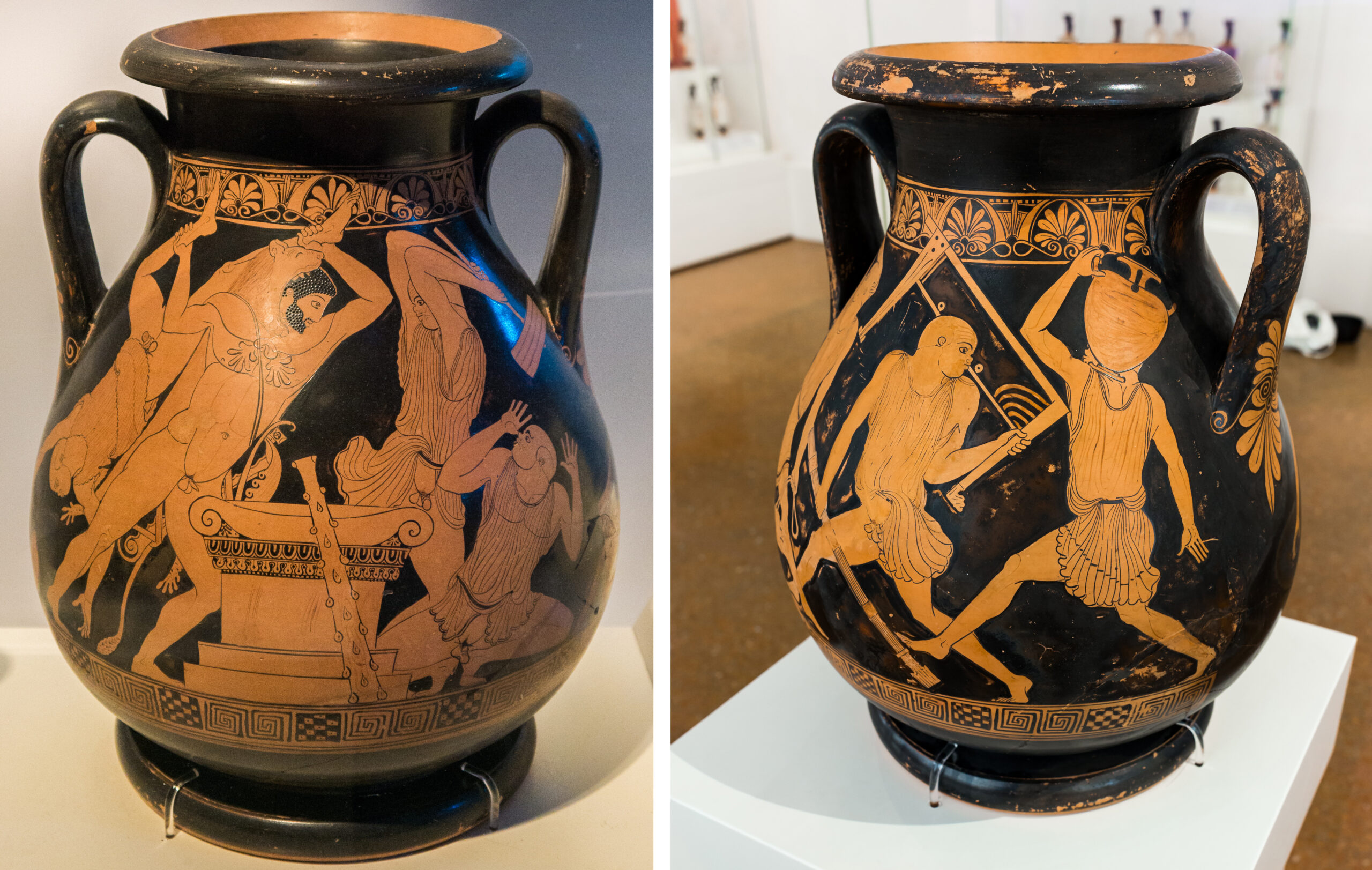The image consists of side-by-side photographs of an ancient Greek amphora, also known as a vase, featuring intricate designs in a light orange hue against a black background. Both photographs primarily focus on the same amphora, capturing it from differing angles to showcase its detailed artwork and structure. 

In the left photograph, the amphora is centered and presents a dramatic battle scene. A man is depicted bending over an altar, gripping another person by the feet, while a figure to his right, brandishing an axe, appears poised to strike. Another figure on the lower right corner, with raised hands, expresses visible fear. 

The right photograph, showing the vase slightly turned, reveals the back side where two additional figures are depicted. One man carries a large piece of wood, and the other balances a similar amphora on his shoulder. Both images highlight the amphora's distinct pear shape and its black handles, which match the vase's black background. 

The vase is adorned with traditional Greek decorative patterns, including the iconic Greek key design at the top and bottom. Together, these images offer a comprehensive view of the ancient amphora's artistic and historical significance, capturing both its front and back depictions.